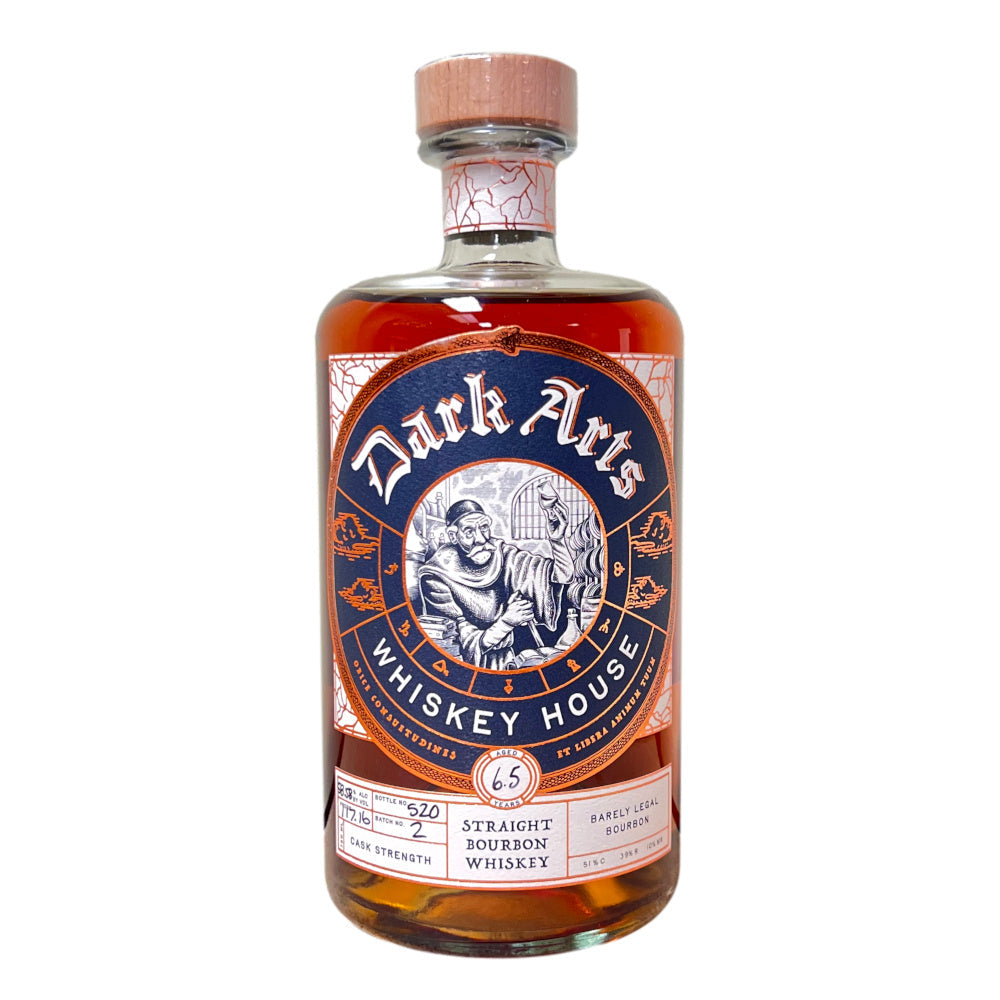The image depicts a full and sealed glass bottle of whiskey, specifically bourbon. The bottle is rectangular with rounded shoulders and features a wooden cork, sealed with plastic wrap. Inside, the bottle is filled with a rich, amber-like brown liquid. The label on the bottle reads "Dark Arts Whiskey House" in a medieval-style, curved white font set against a dark blue background. Below this title, there is a black and white illustration of an old man with white hair, a mustache, and beard, dressed in a robe and holding a glass. This image is centrally placed on the label. Beneath this, additional white text indicates the bottle is labeled "Straight Bourbon Whiskey," accompanied by the phrase "Barely Legal Bourbon." On the left side of the lower label is handwritten batch information, while the right side similarly contains labeling detail. The bottle is pictured against a solid white background with light reflecting off its surface, emphasizing its pristine condition.